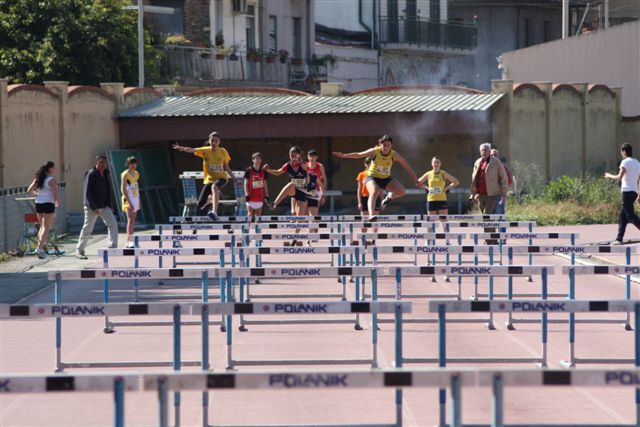This is a daytime photograph capturing a group of young boys and girls participating in a school track and field event, specifically a hurdles race. The athletes, seven in total, are in mid-air as they leap over hurdles positioned on a concrete track, which features black and white markings. Each runner is clad in a yellow tank top with white numbers pinned to their shirts and black shorts, a uniform typically seen in school sports teams. The setting is rich in detail; the weather is sunny, and the background includes a bridge, trees, and a building, which could be part of a campus, an apartment, or a business complex. Additionally, a red shed stands out, possibly serving as a shelter or break area. Observing the scene are people in white and red attire, some walking alongside the track, further suggesting a school event atmosphere. The variety of colors present includes yellow, black, white, red, blue, brown, tan, green, and pink. In the middle foreground, 'Polanic' is visibly marked on the track surface. The image does not contain any date.